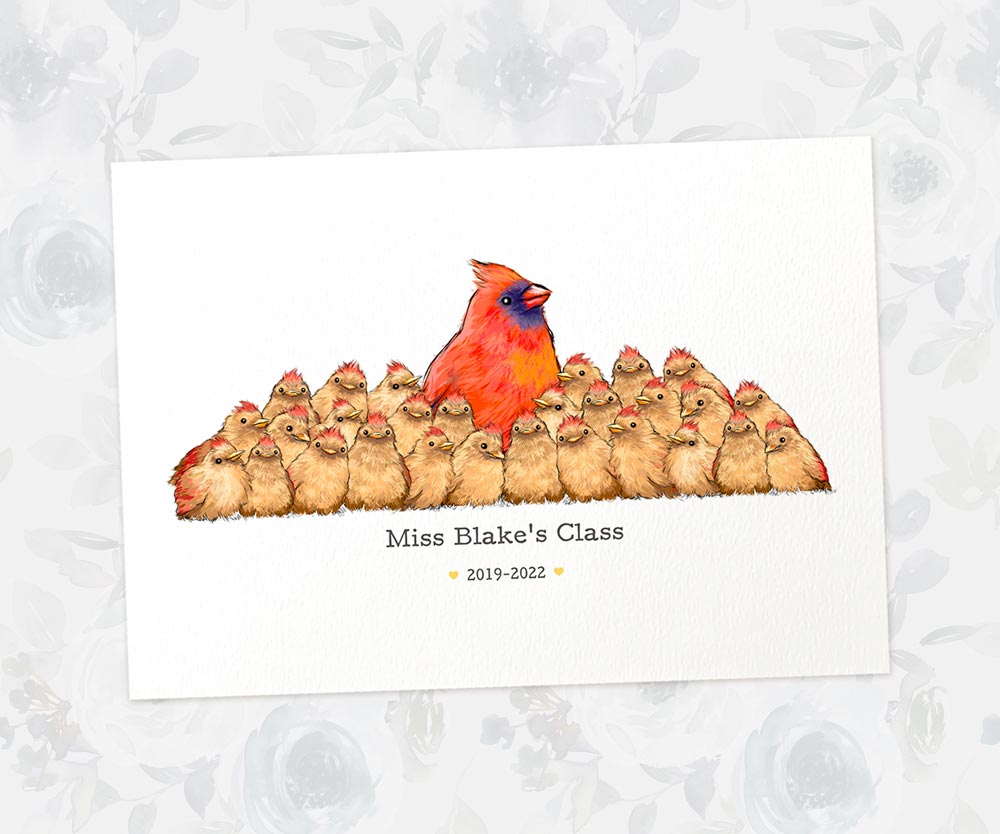In the image, a rectangular white card with grey floral patterns sits on a white surface. In the center of the card is a large, reddish-orange chicken with an orange pointed beak, facing the right. Encircling the chicken's face is a blue ring. Surrounding the larger chicken are numerous baby chicks, approximately fifteen in total, characterized by their yellowish-brown color and small red feathers atop their heads. In elegant text at the card's bottom are the words "Miss Blake's Class 2019-2022," with tiny hearts flanking the date range. The card appears slightly tilted to the left, exuding a casual, handmade charm.